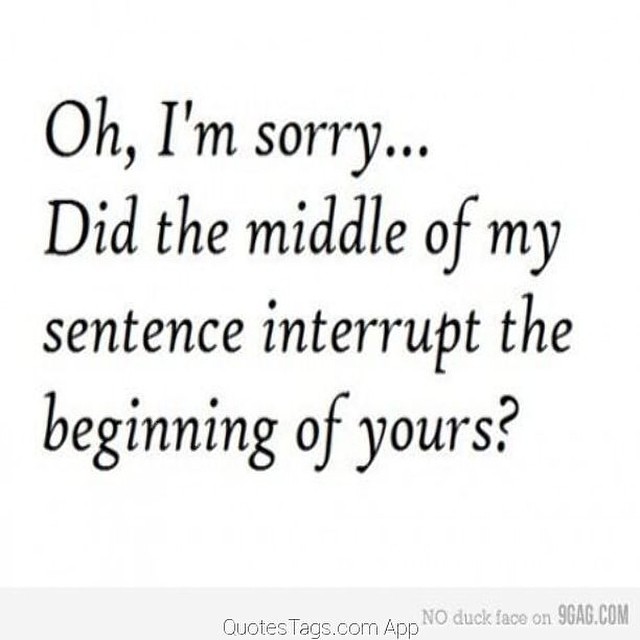The image features a sarcastic quote displayed on a white background with black text that reads, "Oh, I'm sorry... Did the middle of my sentence interrupt the beginning of yours?" The text is in a large, easy-to-read font and arranged in four lines: "Oh, I'm sorry..." on the first line, "Did the middle of my" on the second, "sentence interrupt the" on the third, and "beginning of yours?" on the fourth line. At the bottom of the image, there is a gray banner with text in the center that says "quotes tags dot com app" and some lighter gray text that reads "no duck face on 9GAG.com."